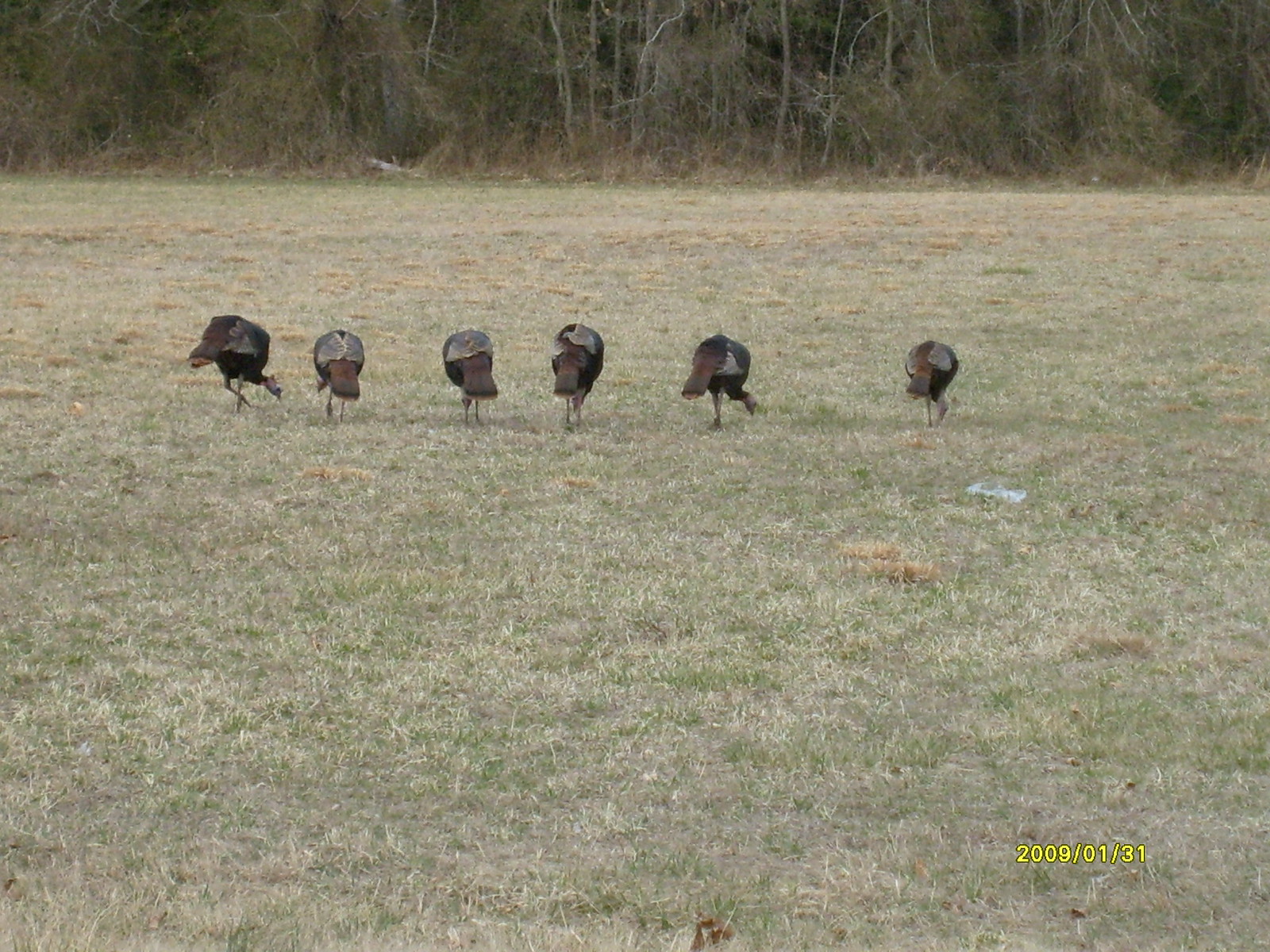In this horizontal daytime photograph, a large, greenish-brown field stretches across the scene. The field is covered in short grass and is bordered in the background by a tree line and bushes with sparse leaves, revealing predominantly brown hues suggestive of the winter season. Six turkeys, primarily dark brown and light brown, stand in a horizontal row at the center of the image. The birds, with their long necks and distinct markings, are mostly facing away, although a couple appear to be pecking at the ground, likely foraging for food. The overall setting is quite open, with the grassy field dominating the majority of the frame, while the wooded area occupies the upper portion of the image. In the bottom right corner, a yellow digital timestamp with a black outline indicates the date 2009-01-31. A small, white object, possibly plastic, is also visible on the grass but does not distract from the primary focus on the turkeys.